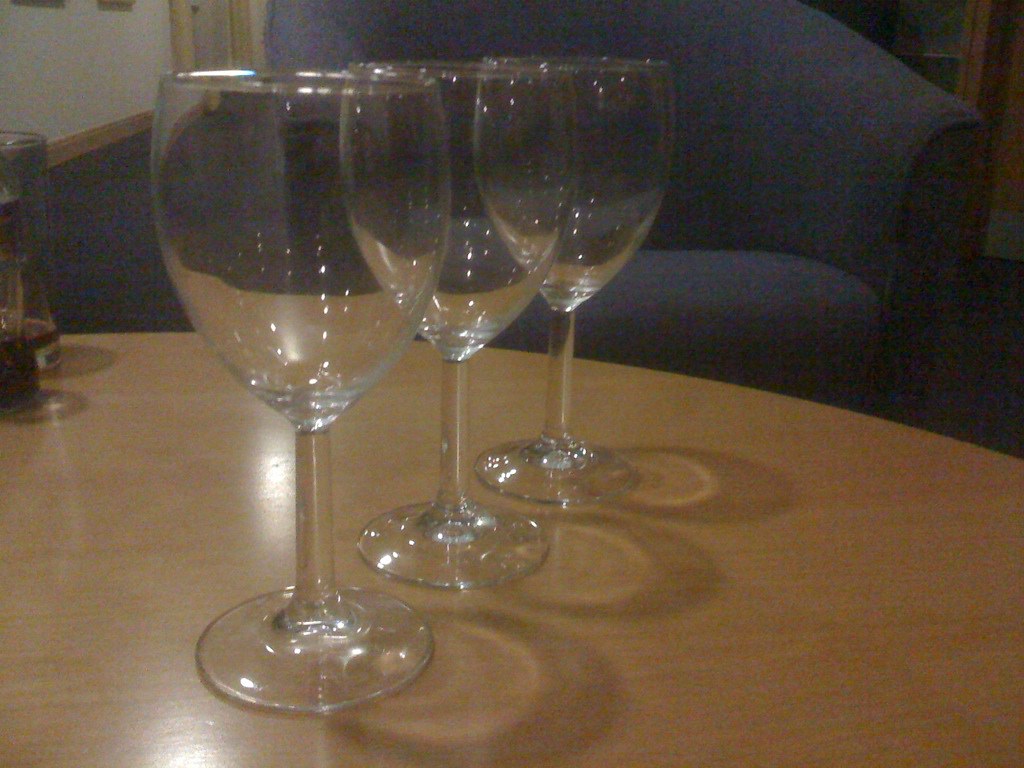This is a low-quality photograph that appears blurred and overexposed, possibly due to poor lighting rather than a camera flash. The image depicts a wooden round table, possibly varnished or featuring a laminate top, with three empty, transparent wine glasses positioned in a slanted row. The glasses are clear and clean, and their shadows create circular patterns on the table’s surface. In the background, there's a plush, possibly suede, navy blue single-seater chair. To the left, partially visible bottles, possibly sauces or dressings, and a whiteboard or chalkboard with a wooden trim can be observed against the white walls of what seems to be an indoor setting. The photograph is neatly cropped to include the entirety of the wine glasses. Despite the blurry and standard definition quality, the essential details of the objects remain discernible.